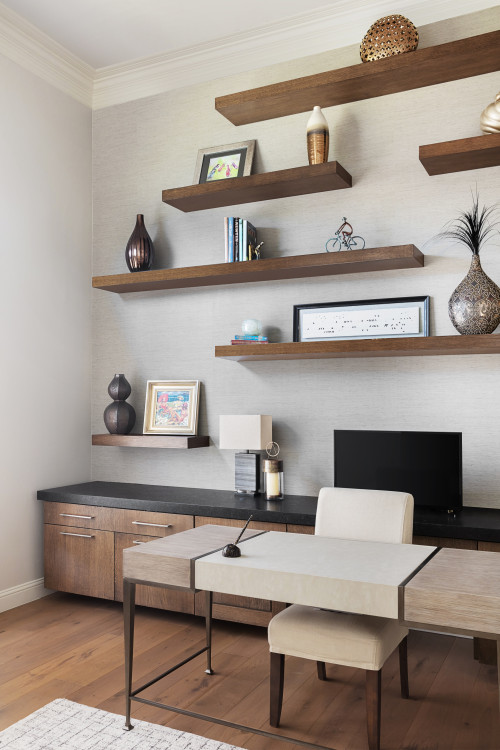The image depicts an elegant and modern home office with a high-ceilinged, white-walled room. The space features hardwood plank flooring in a medium-brown shade, complemented by white trim on the ceiling and baseboards. A wooden desk, consisting of three distinct panels, sits centrally on a white and brown area rug. Positioned beneath the desk is a cream-colored chair with a wooden frame. On the desk is a single item: a pen held upright in a rock-like holder.

Against the far wall, a series of staggered wooden shelves display a variety of decorative items, including vases, a small bicycle sculpture, a framed picture, and neatly arranged books with bookends. Below these shelves, dark brown to light brown cabinets are topped with what appears to be a granite countertop. Centrally placed on this countertop is a flat-screen monitor, possibly a computer or a small television. The room is sparsely but tastefully decorated, following a theme that incorporates shades of brown, black, and white.